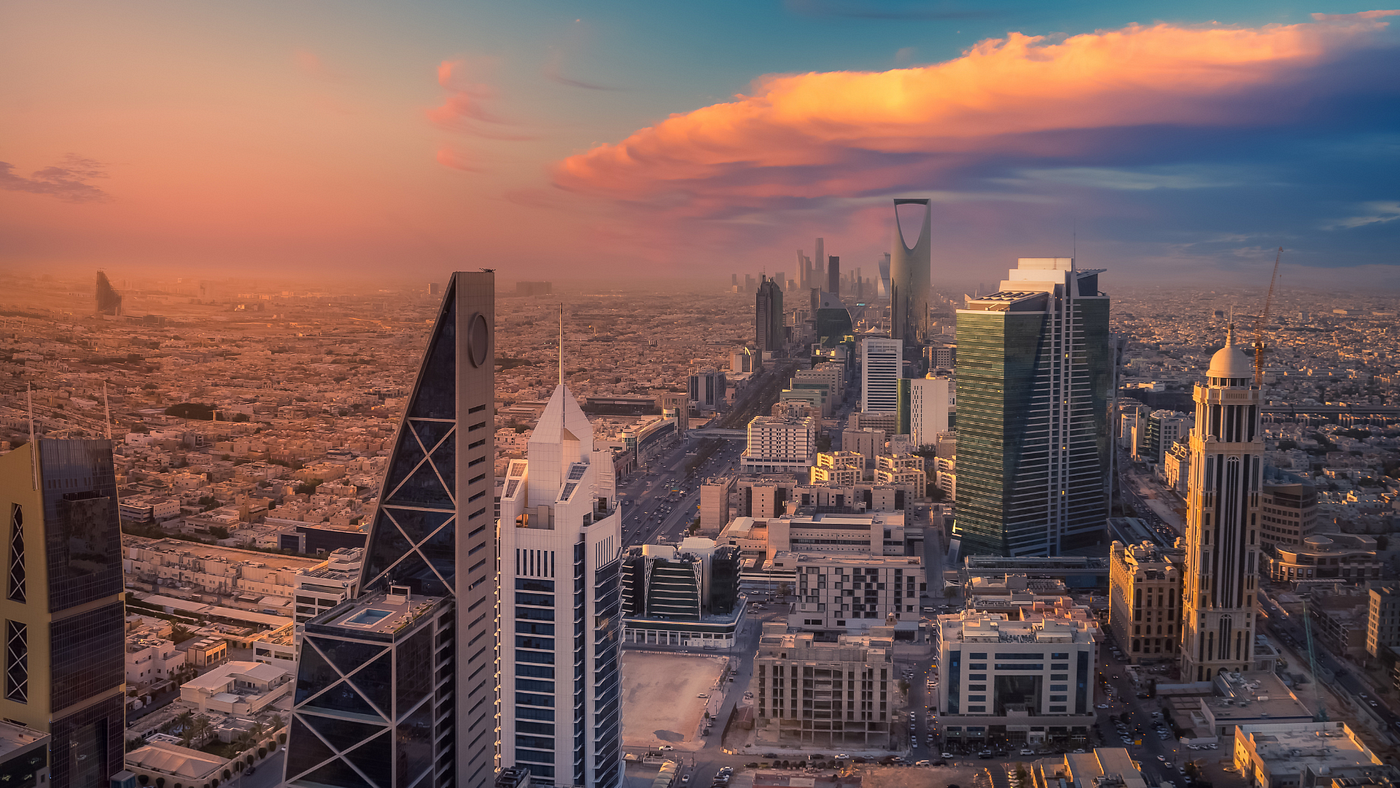This aerial photograph captures a panoramic view of an ultra-modern cityscape, likely taken at sunrise or sunset, given the pinkish clouds and sun glare casting a warm glow across the sky. The overall color palette consists of vivid shades of orange and blue, accented with hints of white, silver, gold, and brown. The city’s skyline features an array of futuristic skyscrapers, diverging from traditional U.S. architecture, suggesting this might be a locale like Abu Dhabi, renowned for its cutting-edge designs.

The foreground is dominated by a striking high-rise with a unique curved shape, where the left side curves inward while the right side remains straight. Another focal point is a distinctive building with a loop or hole near its top, breaking the mold of conventional solid structures. Additionally, a completely white skyscraper with blue windows and a pointed tip stands out, as well as a building topped with a swimming pool. The distant background reveals office buildings with mirror-like windows, contributing to the overall modern aesthetic. Streets weave through the urban landscape below, while a slight haze on the horizon enhances the sense of scale and depth.